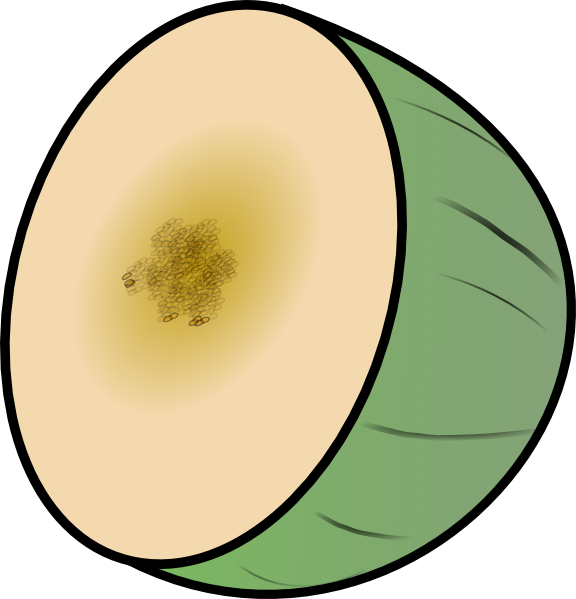The image depicts a digital illustration of a melon that has been cut in half. The illustration features a white background with the melon outlined in black. The outside of the melon is green with black stripes, giving it a watermelon-like appearance. The inside of the melon is divided into concentric sections of color: just inside the black outline, the flesh of the melon starts as a tannish peach color, progressing to a darker yellow hue toward the center. The seeds are depicted as small, round brown and black circles, layered on top of each other toward the middle of the fruit. The entire illustration is rendered with clear, simple lines, emphasizing the shape and ridges of the melon while maintaining a clean, digital aesthetic.